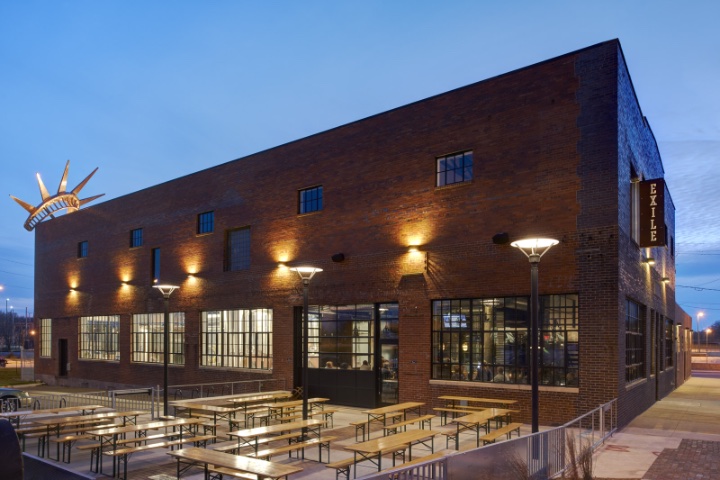The photograph captures a rectangular, two-story commercial building constructed from red bricks, identifiable by its signboard that reads "Exile" in bold letters. The building, likely repurposed from a factory into a bar or a restaurant, features large windows with black frames on the bottom floor and a glass door, allowing a view inside where patrons are visible under illuminated lights. The sky, transitioning from day to night, casts a subdued blue hue, complemented by the exterior lights that lend a warm glow to the scene. Prominently, the top-left corner of the building boasts a crown resembling the one on the Statue of Liberty, adding a distinctive character that suggests an American locale. The outdoor patio, surrounded by a gray-painted railing, is equipped with numerous benches and tables for seating. Despite the inviting arrangement, the patio remains unoccupied, and the surrounding area appears sparse and dry, with few neighboring structures.